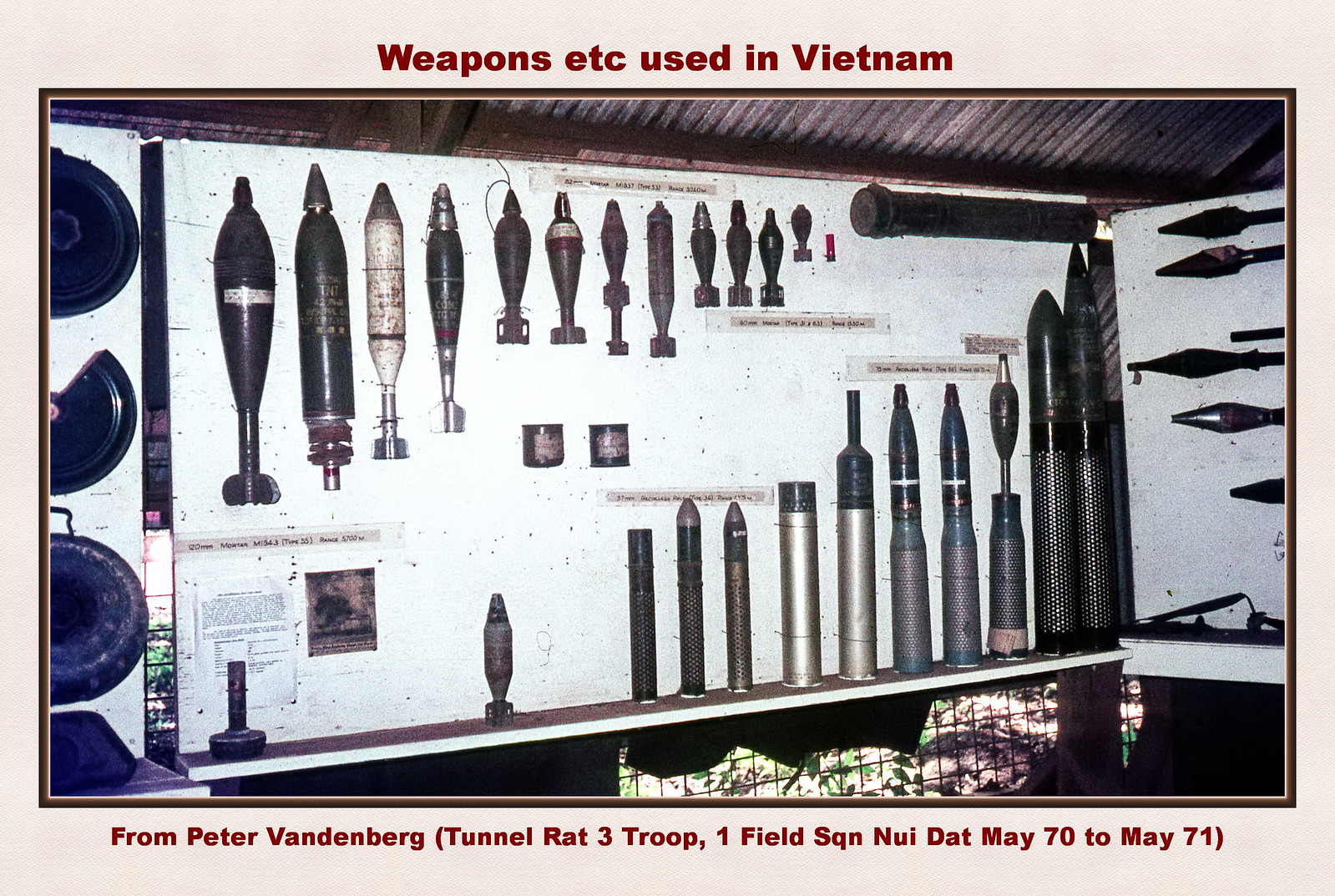This photograph, set in a landscape orientation with a light tan border, showcases a meticulously arranged display of weapons used in the Vietnam War. The top center of the image features a bold red caption reading "Weapons etc. used in Vietnam." Mounted on a whiteboard attached to a wire mesh wall, likely within a shed or similar structure, the display includes a diverse array of bombs, missiles, bullets, and incendiary devices, varying in size from several feet to just a few inches. Above the display, a tin roof is visible, adding to the rustic setting. Below the weapon exhibit, another red text reads, "From Peter Vandenberg (Tunnel Rat 3 Troop, 1 Field Sqn, Nui Dat, May 70 to May 71)," providing context and attribution for the collection.